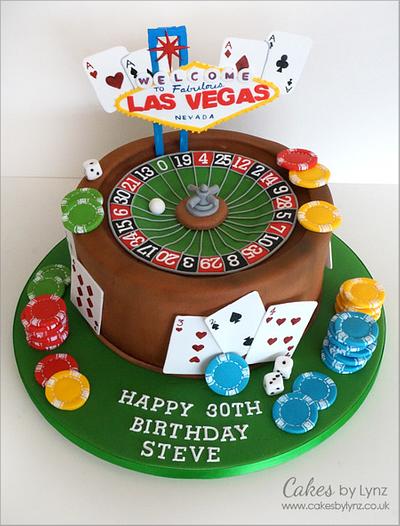This rectangular image, encased in a thin gray border, showcases a celebratory cake meticulously crafted by Cakes By Lins. The upper third of the background is a light gray wall that transitions into a darker gray for the remaining two-thirds. In the lower right-hand corner, "CAKES BY LINS" is elegantly written in gray cursive and print, followed by the website www.cakesbylins.co.uk.

At the center of the image lies a stunning cake, approximately two layers and circular in shape, adorned in brown fondant. The cake's base is decorated with a green circle featuring white text that reads "Happy 30th Birthday, Steve." Surrounding the cake are colorful poker chips in green, red, yellow, and blue. At the front, there are playing cards adding to the casino theme, while the top of the cake boasts a detailed roulette wheel complete with a tiny white ball and additional poker chips on the corners. Dominantly displayed at the back is a sign replicating the iconic "Welcome to Fabulous Las Vegas, Nevada" sign, flanked by the four ace poker cards emerging from both sides. 

This visually rich and detailed cake is clearly designed for a casino-themed celebration, encapsulating the glitz and excitement of Las Vegas.